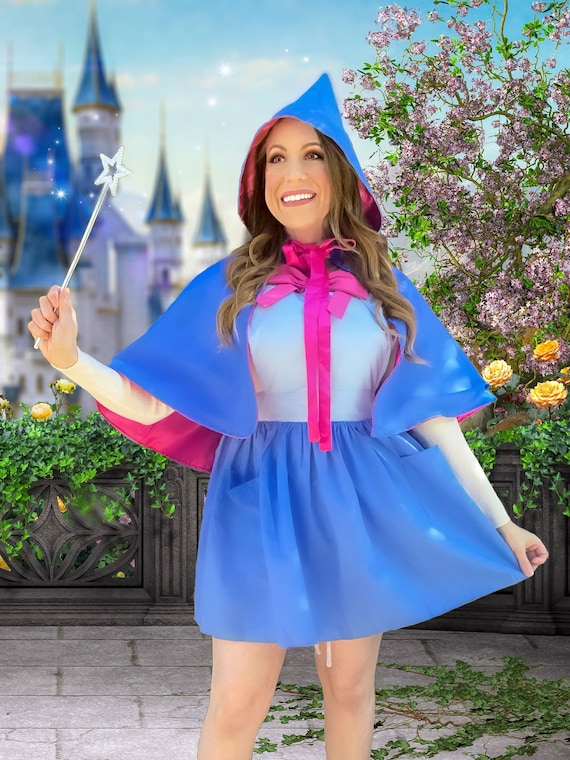In a vibrant and whimsical scene, a woman dressed as a fairy godmother stands gracefully in the foreground, smiling warmly. She is framed by an out-of-focus castle with striking blue peaks under a clear blue sky. The backdrop is adorned with colorful flowers and lush foliage, including large yellow roses and a variety of pink blossoms, alongside a green tree with purple buds. A brown waist-high fence and a stony ground interspersed with greenery add to the picturesque setting.

The woman herself is the epitome of enchantment, wearing a blue hooded cape that is strikingly lined with bright pink fabric. This pink hue is echoed in the bow tied neatly under her chin. Her outfit comprises a light blue shirt coupled with a darker blue skirt that falls above her knees, mirroring the cape's rich blue hue. Her long brown hair flows gracefully, complementing her fair to medium complexion and brown eyes. In her right hand, she delicately holds a silver wand topped with a glittery silver star, adding a touch of magic to this captivating and joyful photograph.